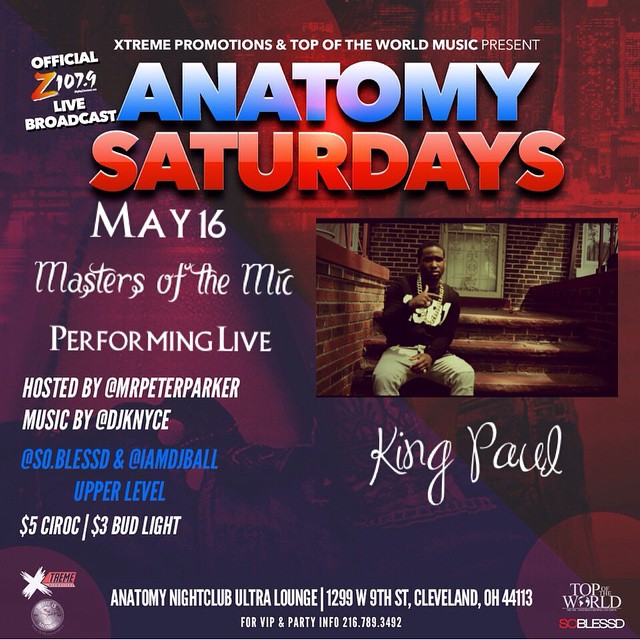The advertisement is a vivid promotional leaflet likely distributed to the public, showcasing an upcoming event at the Anatomy Nightclub Ultra Lounge. The event, dubbed "Anatomy Saturdays," is scheduled for May 16th and is presented by Extreme Promotions and Top-of-the-World Music. It features a live performance by the "Masters of the Mic," hosted by Mr. Peter Parker. The musical lineup includes DJ Nice, So.Blessed, and DJ Ball. Attendees can enjoy drinks with special offers: $5 Ciroc and $3 Bud Light.

The image backdrop consists of a faded cityscape in red hues, accentuating the bold event details. Prominence is given to "Anatomy" rendered in blue, while "Saturdays," "May 16th," and other key details stand out in contrasting colors. Notably, there is a photo of a musician, presumably a performer at the event, seated on brick steps donning a black long-sleeve shirt with the year "1987" in white, white pants, and a gold chain, throwing a hand symbol, against the backdrop of a brick house. Below this image, "King Paul" is inscribed in elegant cursive.

Additional elements include logos such as the official Z107.9 Live Broadcast. For those seeking VIP and party information, the advertisement provides the phone number 216-789-3492. The venue is located at 1299 West 9th Street, Cleveland, Ohio, 44113.